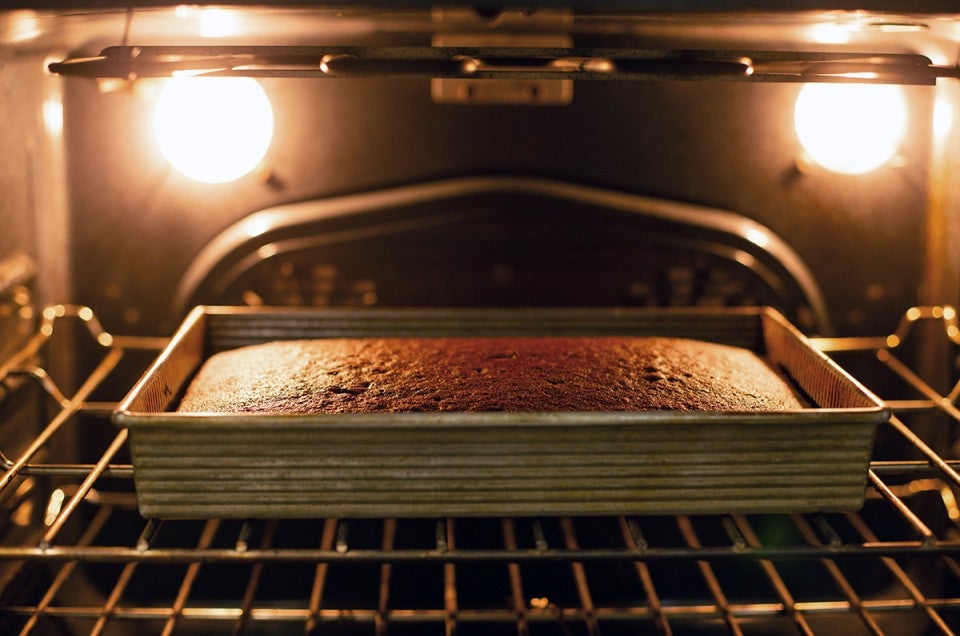A black-and-white photo captures the inside of an oven with two shelves. The oven door is open, revealing a heating element suspended from the top. On the top shelf sits a well-used square metal baking pan containing a perfectly baked dessert, possibly a cake, banana bread, or brownies, with a beautifully browned top. The oven lights, situated in the top corners, are on and their reflections can be seen along the sides of the oven, illuminating the scene. The racks, though a bit dirty, add authenticity to the image. The dessert appears just finished and ready to be removed, still potentially hot from baking.